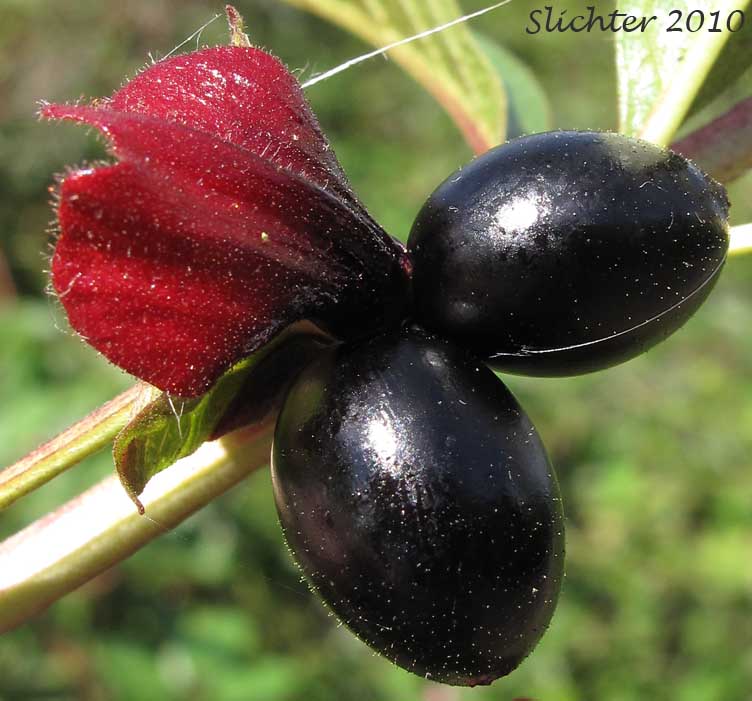This photograph features a striking close-up of a unique flower against a muted, faded green background of grass, emphasizing the natural setting. Dominating the image are two dark, grape-shaped pods, almost black in color, one angled towards 2 o'clock and the other towards 4 o'clock. These pods are attached to a deep red, almost succulent-like petal adorned with tiny needle-like hairs, which convey a fuzzy texture. The flower's intricate details are enhanced by green stems, some of which display a shiny gold tint, extending from the bottom left corner. Notably, the name “Slichter 2010” appears prominently in the top right corner, identifying the image.